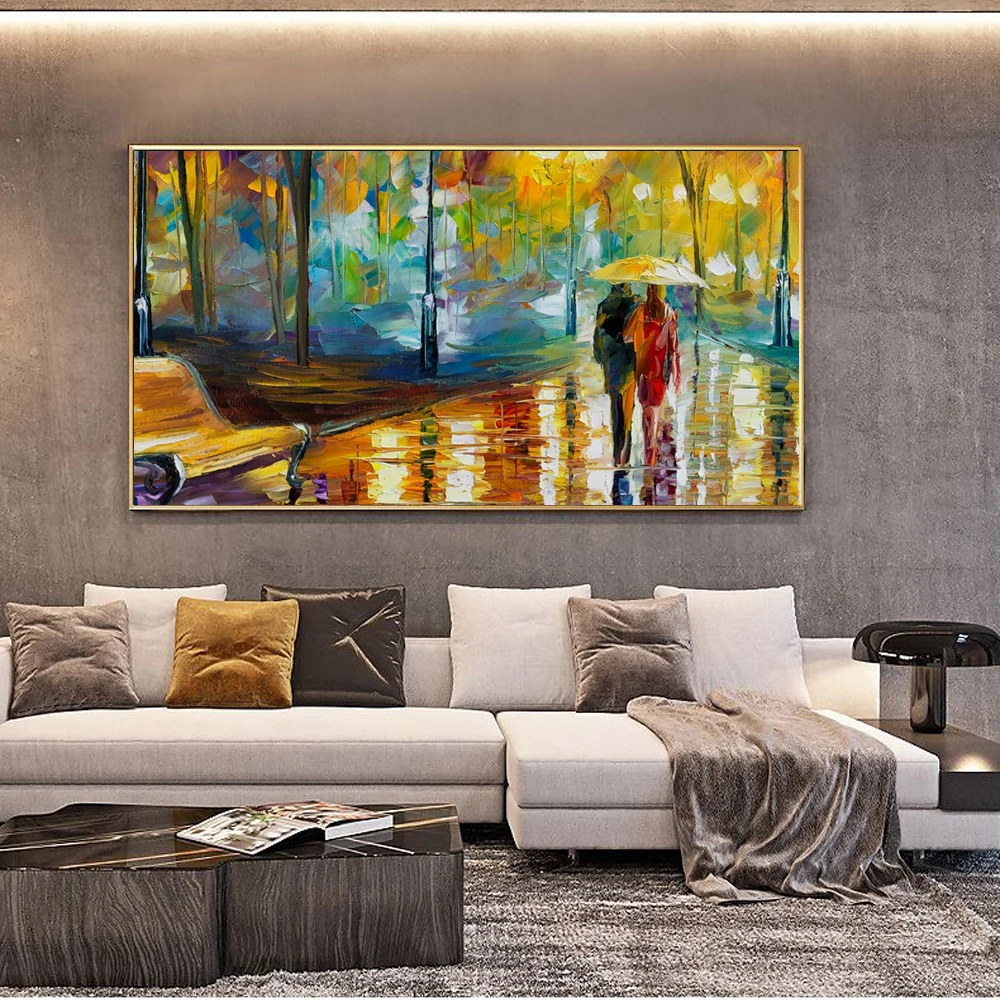This photograph depicts a modern living room featuring a textured matte gray wall that gives the space a contemporary yet subtle backdrop. Dominating the room is a spacious, white sectional sofa with a chaise lounge on one end. The sofa is adorned with an array of pillows in neutral tones including silver, gold, white, black, brown, and gray. Draped over the chaise lounge is a cozy gray blanket that matches one of the pillows. 

At the center of the living room is a wooden coffee table with a black glass top, featuring a distinctive wood grain pattern and a book placed neatly on it. A plush carpet in shades of gray and white covers the floor, complementing the overall neutral palette. To the right of the sofa stands an end table with a sleek black lamp, adding a touch of modern elegance.

Hanging prominently on the gray wall is a large, vibrant painting that captures the eye with its dynamic use of colors and reminiscent style of Van Gogh. The artwork depicts a rainy scene where a man and a woman walk under a yellow umbrella along a path made of orange and white, reflecting the shimmering rain. To the left, there's a park bench, and in the background, tall trees with blotches of green, blue, yellow, and red leaves create a blurred, almost whimsical landscape. The painting’s vivid hues stand in stark contrast to the muted tones of the living room, creating a striking focal point within this stylish, modern space.